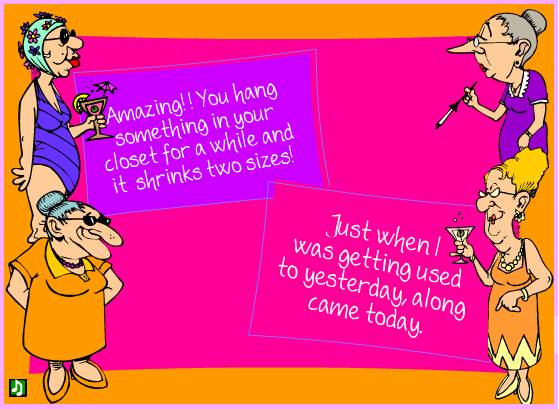This cartoonish, brightly colored image features a humorous depiction of four elderly women, each positioned in one of the corners of the image. The overall aesthetic is predominantly pink with an orange border, and the background features exaggerated, cartoon-like illustrations.

In the upper left corner, a woman in a blue one-piece bathing suit and swim cap enjoys a cocktail. In the lower left corner, a woman with a large nose, blue hair, and an orange dress looks on. The lower right corner depicts another woman clad in an orange dress, holding a cocktail glass, with gold-colored hair styled in an elegant updo. In the upper right corner, a woman with green hair, a pointed nose, and a purple dress holds a long cigarette holder. Each woman sports a distinct, quirky style, adding to the humor of the scene.

The pink background features two slanted signs with witty captions. The upper sign reads, "Amazing. You hang something in your closet for a while and it shrinks two sizes." Meanwhile, the lower sign says, "Just when I was getting used to yesterday, along came today." This delightful image, suitable for a card or social media post, captures the comedy and camaraderie among friends with its amusing characters and catchy phrases.